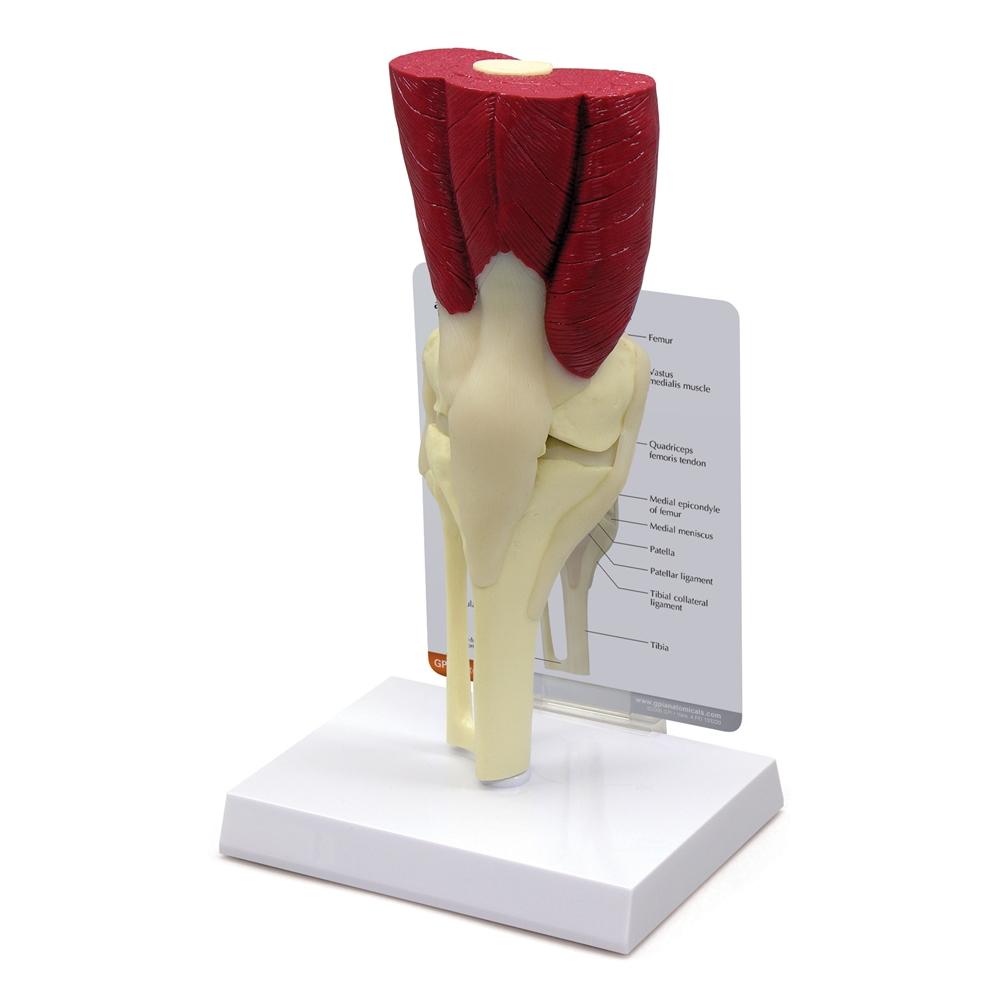This image is a detailed photograph of a 3D anatomical model you would find in a doctor's office, particularly in the office of a physical therapist or orthopedist. The model, which is a replica of a human knee joint, stands upright on a shiny, white plastic base. The knee model itself features various components, including bones, muscle, cartilage, and the patella ligament. On top of the bone are four sections highlighted in red, indicating different important areas. Behind the knee model, there is an upright white chart with black lettering. This chart provides a detailed diagram of the knee, listing specific anatomical landmarks such as the femur, quadriceps femoris tendon, patella, and tibia, with lines pointing to these parts on the model. The upper corner of the chart has an orange background, adding a touch of color to the otherwise clinical presentation. This setup is designed to help doctors explain the intricacies of knee anatomy to their patients.